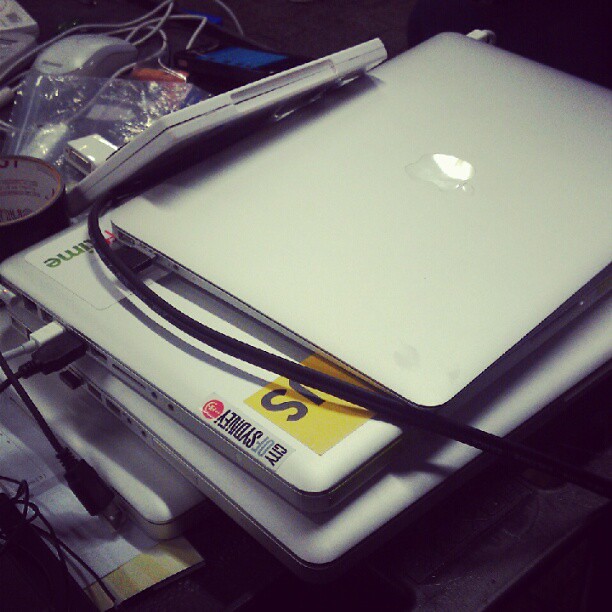The image depicts a cluttered desk or workspace featuring a stack of four electronic devices, likely laptops or tablets, with detailed observations of each device and surrounding items. The top device is a modern Apple MacBook, recognizable by its sleek silver design. Beneath it, the second device, also silver, has several stickers: a partial yellow sticker, a white sticker obscured at the bottom, and a visible side sticker reading "City of Sydney." Two cords, one white and one black, are plugged into one of these devices, with an additional black cord hanging down. The background reveals assorted computer accessories and clutter, including a wired mouse, a partially used roll of black duct tape, a Ziploc bag, a white media case potentially for CDs or DVDs, and various cables. A black box with blue accents is also visible amidst the disarray, contributing to the overall sense of a busy and disorganized workspace.